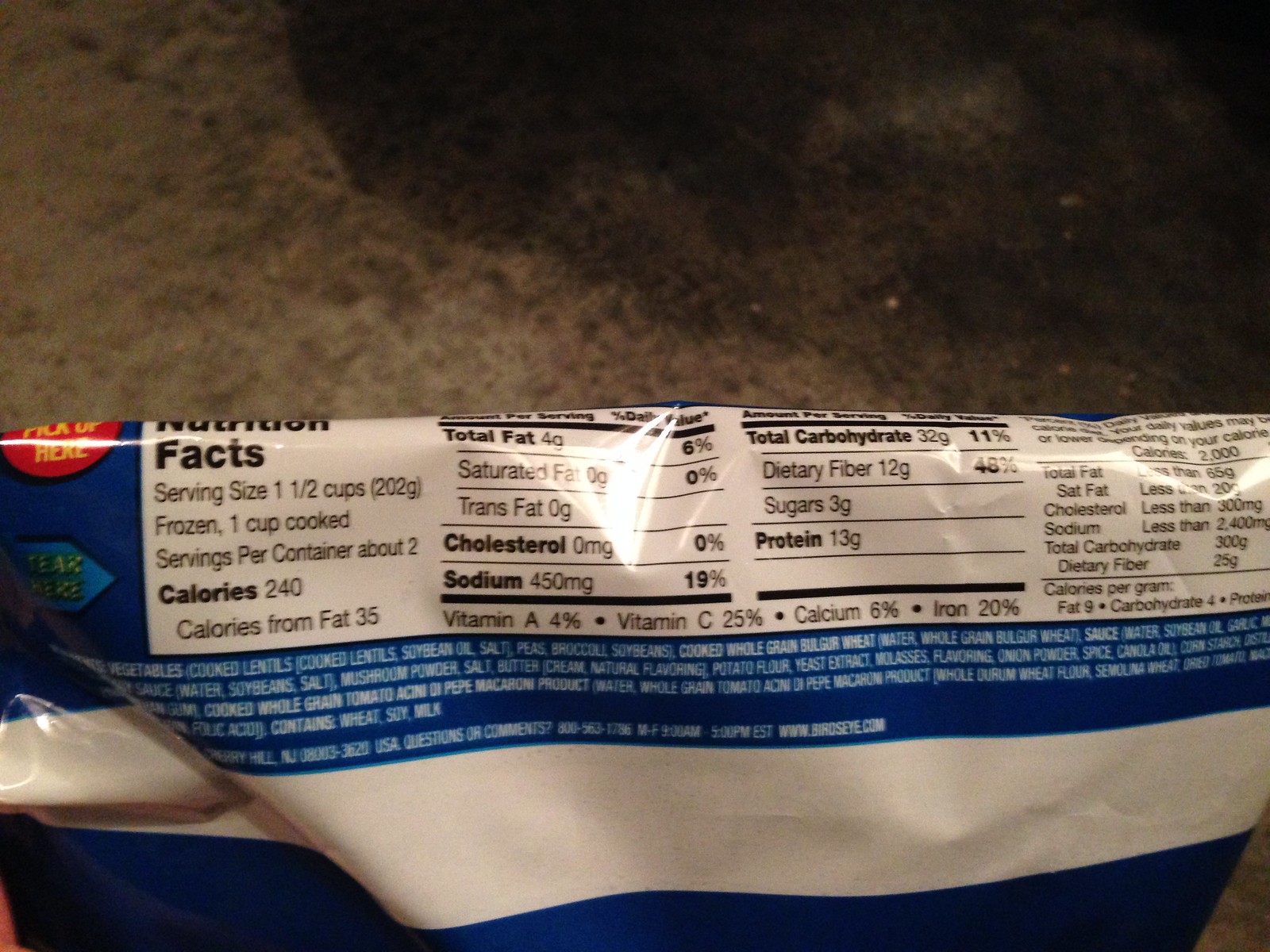The photograph captures a blue and white plastic food packaging, likely for frozen vegetables, lying on a surface that appears unclean, possibly a dirty carpet or outdoor area with visible debris. The image is taken indoors. The bag is folded over at the top, revealing a detailed nutrition facts label. The label states that the serving size is 1.5 cups frozen or 1 cup cooked, with approximately two servings per container. It details the nutritional content, including 240 calories (35 from fat), 4 grams of total fat, 0 cholesterol, and other nutritional information. The ingredients listed include peas, broccoli, and soybeans. The packaging also features instructional text near the fold: a red dot with "pick up here" written in yellow and a blue arrow with "tear here" in green.